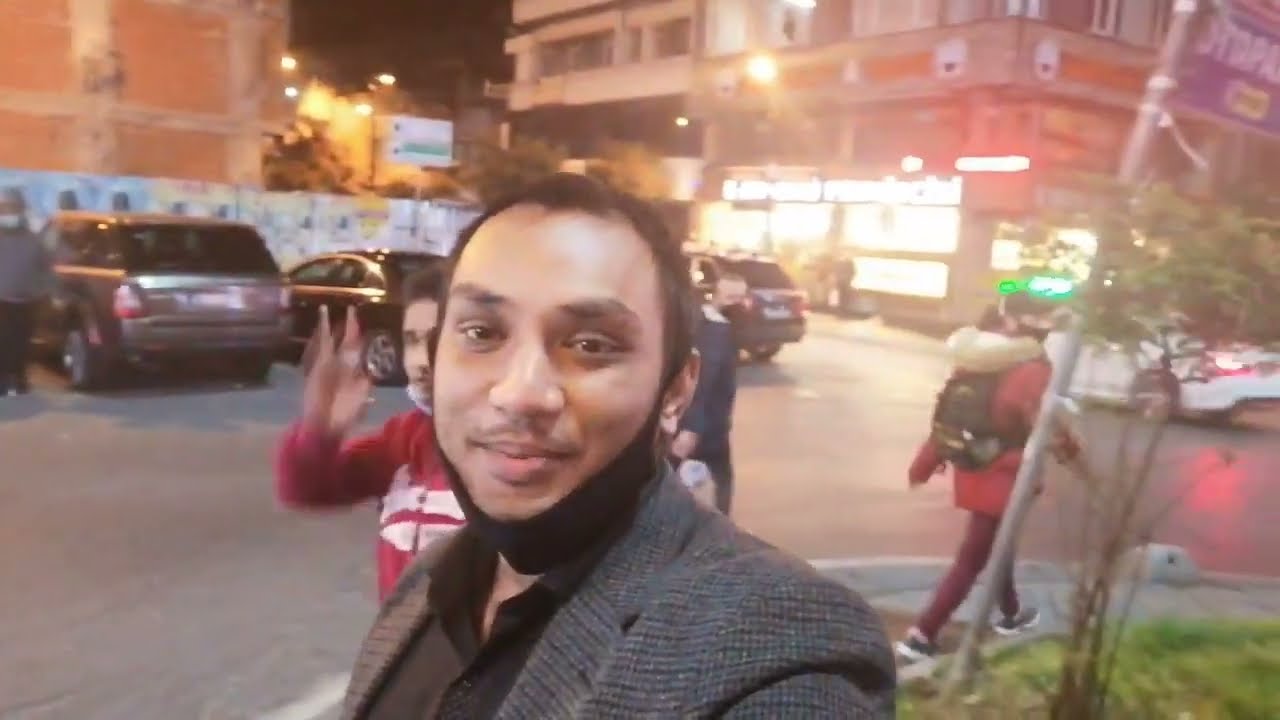In the photo, a young Latino man in his early to mid-20s, with dark hair, dark eyebrows, and a mustache, is taking a selfie on a nighttime urban street. He is wearing a black button-down shirt with a collar, topped with a gray tweed suit coat. His COVID mask is pulled down below his chin, creating the illusion of a beard. The young man is smiling into the camera, his arm outstretched to capture the shot. Behind him, a busy street scene unfolds: people are walking up and down the street, including a young man in a red hoodie who appears to be waving at the camera. There is a parking lot with several parked cars and a metal pole with an indecipherable blue sign. Tall buildings with well-lit windows frame the background, enhancing the urban atmosphere. Over his left shoulder, a young woman in a red parka jacket and maroon leggings walks along the sidewalk. The composition captures the lively essence of a city at night, filled with movement and light.